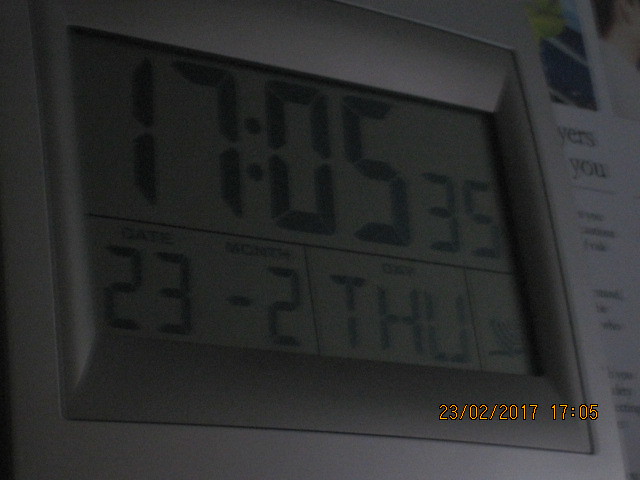A detailed close-up photograph of a clock device's screen displaying time and date information. The top section of the screen shows the current time in a 24-hour format, reading 17:05:35, which corresponds to 5:05 PM. The lower left corner of the screen is segmented into three squares, with the first two indicating the date as the 23rd of February, suggesting a non-American date format. The display also notes that the current day is Thursday. The third square is not clearly legible. A timestamp is visible at the bottom right corner of the image, marking the photo as taken on the 23rd of February, 2017, at 17:05.